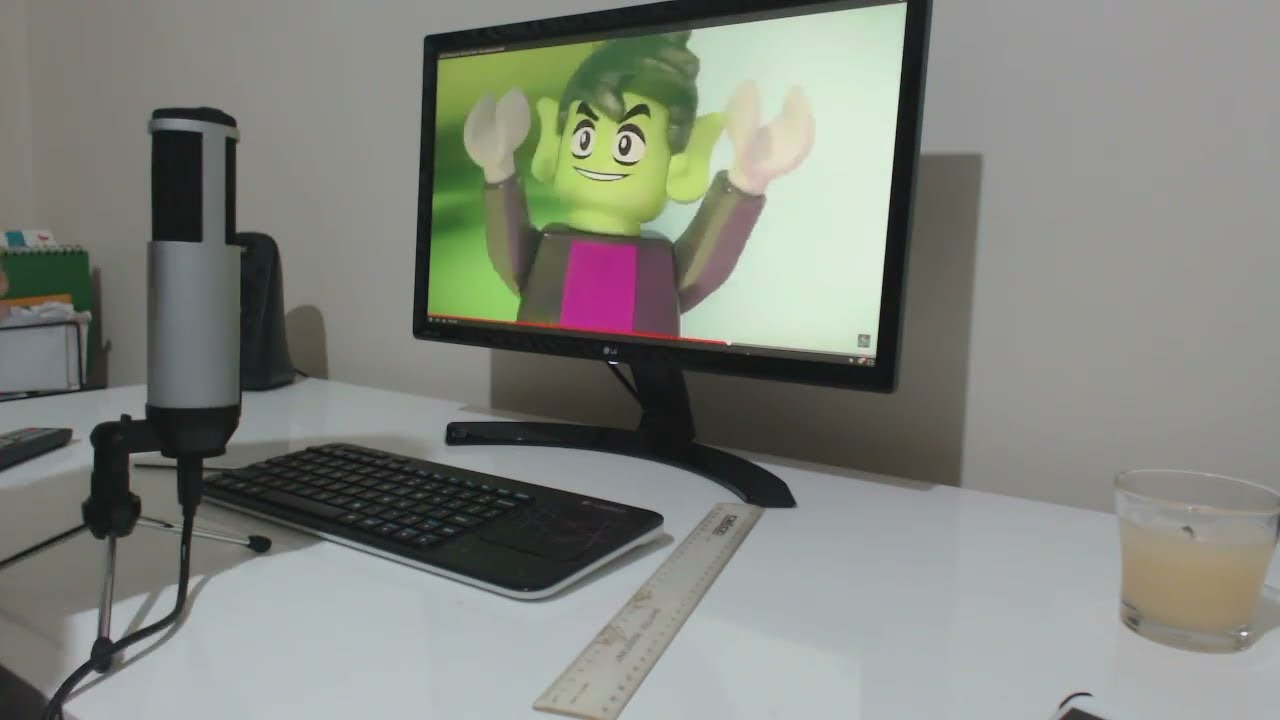The image depicts a detailed scene of a workspace, featuring a person engaged with a computer on a neatly organized white desktop. The upper half of the image showcases a light gray wall forming the background, while the lower half is dominated by the pristine white surface of the desk. At the center of this scene is a black computer monitor displaying what appears to be a video or movie titled "Bigger Stories." The screen prominently features big white letters spelling out the title, accompanied by a full moon in the upper right corner, against a backdrop of a dark cityscape with buildings illuminated by glowing yellow lights. Additionally, there's a visible red progress bar at the bottom of the screen, indicating the video’s duration.

A black keyboard is placed directly in front of the monitor, and to its right, a large silver rectangular ruler rests on the desk. Just beyond the keyboard, on the far right, sits a clear glass jar holding a light brown or peach-colored candle. The left-hand side of the image is occupied by the person's right hand and forearm, which appear to be resting on the table. The individual is wearing a maroon leather jacket. Also noticeable is a glass containing some form of liquid, perhaps an alcoholic drink, positioned nearby on the desk.

The setting creates the impression of an office or a personal workspace, with the individual seemingly watching a video on their desktop while surrounded by a few distinct items, including the ruler and the candle. The overall ambience hints at a comfortable yet focused environment for either work or leisure.